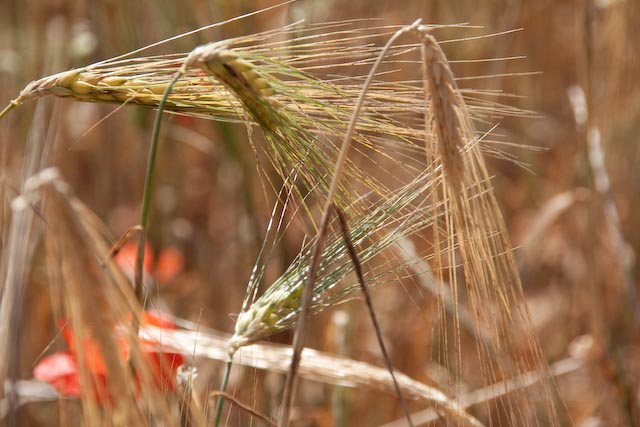This close-up photograph captures a detailed view of sparse, dying grasses or straw-like plants. The three main plants in the foreground display thin bases characterized by a mix of muted browns, tans, and occasional hints of green. The delicate, slender stalks appear to be folding or bending over, suggesting they may be parched and in need of water. The sparse foliage at the tips possesses a subtle blend of light green, yellow, and brown hues.

In the background, a blurry, indistinct field of similar grasses extends, awash in a sea of muted browns and indistinct shapes, contributing to a sense of desolation and dryness. Adding a touch of color and mystery, a bright orange element—perhaps a flower or some other noticeable object—appears in the lower left-hand corner, though its exact nature remains unclear due to the blur.

The entire scene, photographed in a forest or woodland setting, evokes a sense of arid decay, with the withered grasses almost breaking off their stalks, and the landscape behind shrouded in an unfocused haze of additional dying flora.